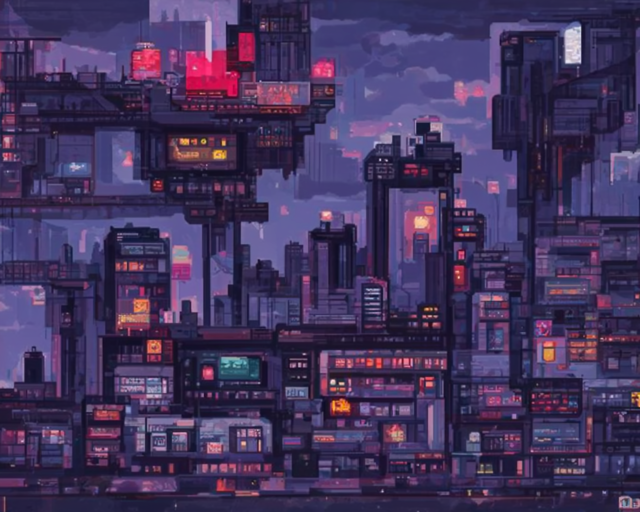The image is a highly detailed pixel art depiction of a cyberpunk cityscape, presented in landscape orientation. The scene is densely packed with a mix of buildings varying in height. In the foreground, there are shorter buildings, each under ten stories tall and tightly built next to one another, displaying brightly lit windows in shades of red, orange, and yellow. On the left side of the foreground, there is a particularly notable building with a red construction feature on its balcony.

As the eye moves towards the background, the cityscape transitions to include much taller skyscrapers, culminating in a colossal building situated on the top left of the image. This massive structure features a two-level platform, with additional buildings on its upper portion adorned with red banners. Partially visible on the bottom left is a large structure with golden interior lights and a bridge that is cut off from full view. Positioned near the left side of the image, a mounted TV screen emits a green hue.

Dominating the top right portion of the image is another tall building, equipped with platform-like structures at its summit. Notably, the image maintains its clean, intricate pixel art style, even though it appears slightly blurry, suggesting it was likely enlarged from a smaller original. Overall, this cyberpunk cityscape exudes a dystopian atmosphere, amplified by its vivid colors and intricate design elements.